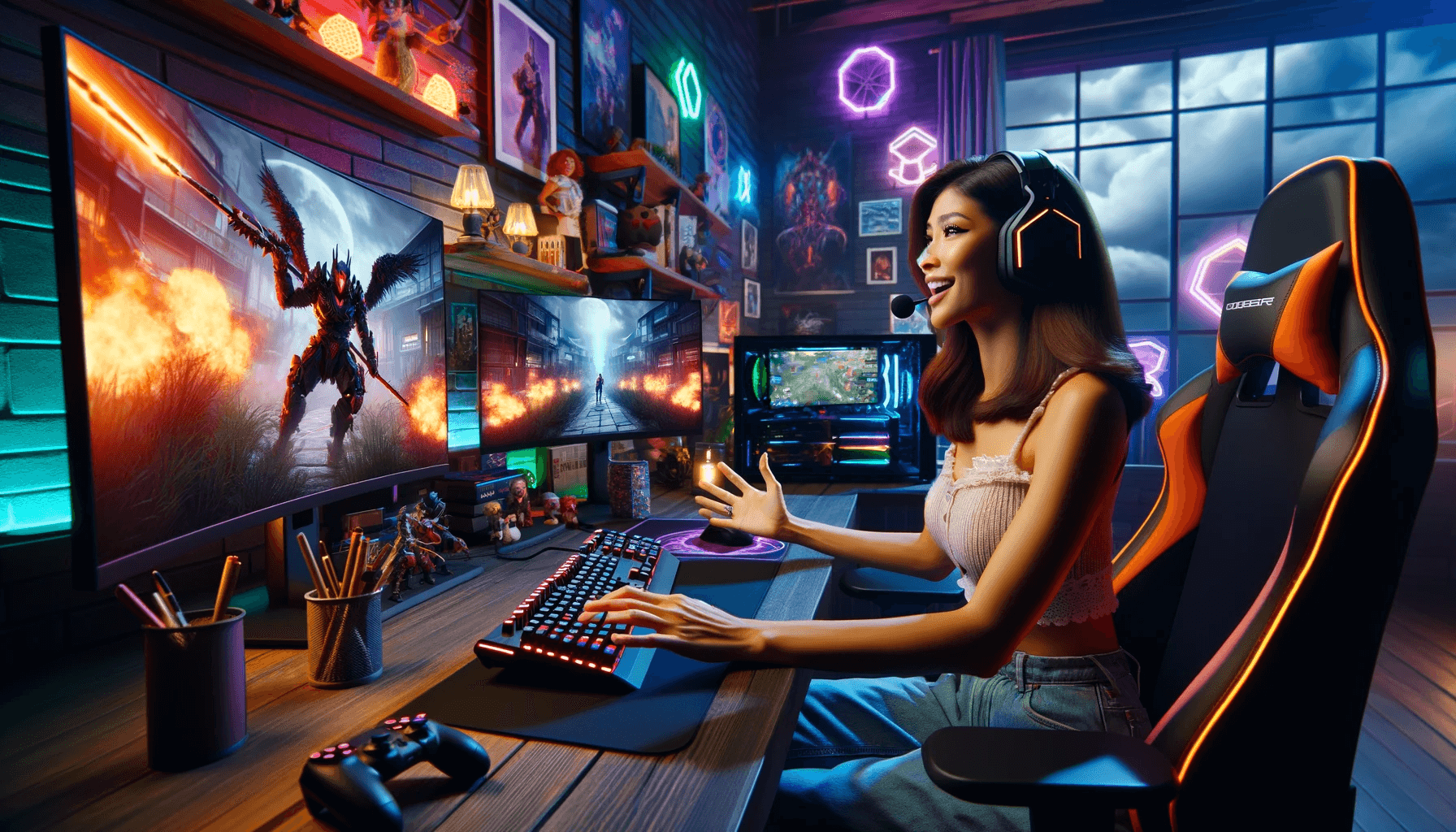The image portrays a young Asian woman with long, straight, dark hair, sitting in a black and orange gamer chair, engrossed in playing a video game. She is wearing black and orange headphones with a microphone, a pink crop top with spaghetti straps, and blue jeans. The scene captures her seated at a large wooden desk with a black keyboard and a video game controller nearby. Her desk is cluttered with several cans holding pencils and figurines. She is smiling and looking at a primary computer monitor which displays a winged monster amidst a fiery street scene, while a second monitor shows a similar gaming scene. The surrounding room features black and purple walls adorned with neon decorations, posters depicting fantasy gaming scenes, and LED lights. The room's large window, framed by long drapes, reveals a cloudy night sky illuminated by distant lights. The woman appears excited and fully immersed in the game.